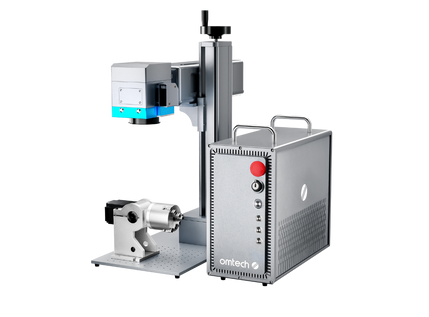This image portrays a sleek, modern piece of lab or industrial equipment, predominantly metallic and silver in color, set against a stark white background. The central component is a rectangular, silver-gray box resembling a computer tower, featuring the brand name "Arctec" (or possibly "Odd Tech") on its surface. The front of the box is detailed with several black dots, potentially indicating keyholes or ventilation, along with a prominent red knob at the top left and additional smaller black knobs below it. Grating or vents are visible on the sides for ventilation, and two silver handles are situated on the top.

Extending from the left side of this box is a tall, movable metal arm equipped with what seems to be an adjustable mechanism. This arm supports a cross-section that includes a lens or microscope, identified by a black circular lens pointed downwards. Some colored bands—light green and dark blue—adorn the lower part of this structure, which also features a blue section near the base. The apparatus includes additional cylindrical and frame-like components fixed to the base, suggesting functionality similar to laboratory or industrial diagnostic equipment. The intricate design and various adjustable parts imply that this machine could be involved in precision tasks such as 3D printing, etching, or other detailed technological processes.